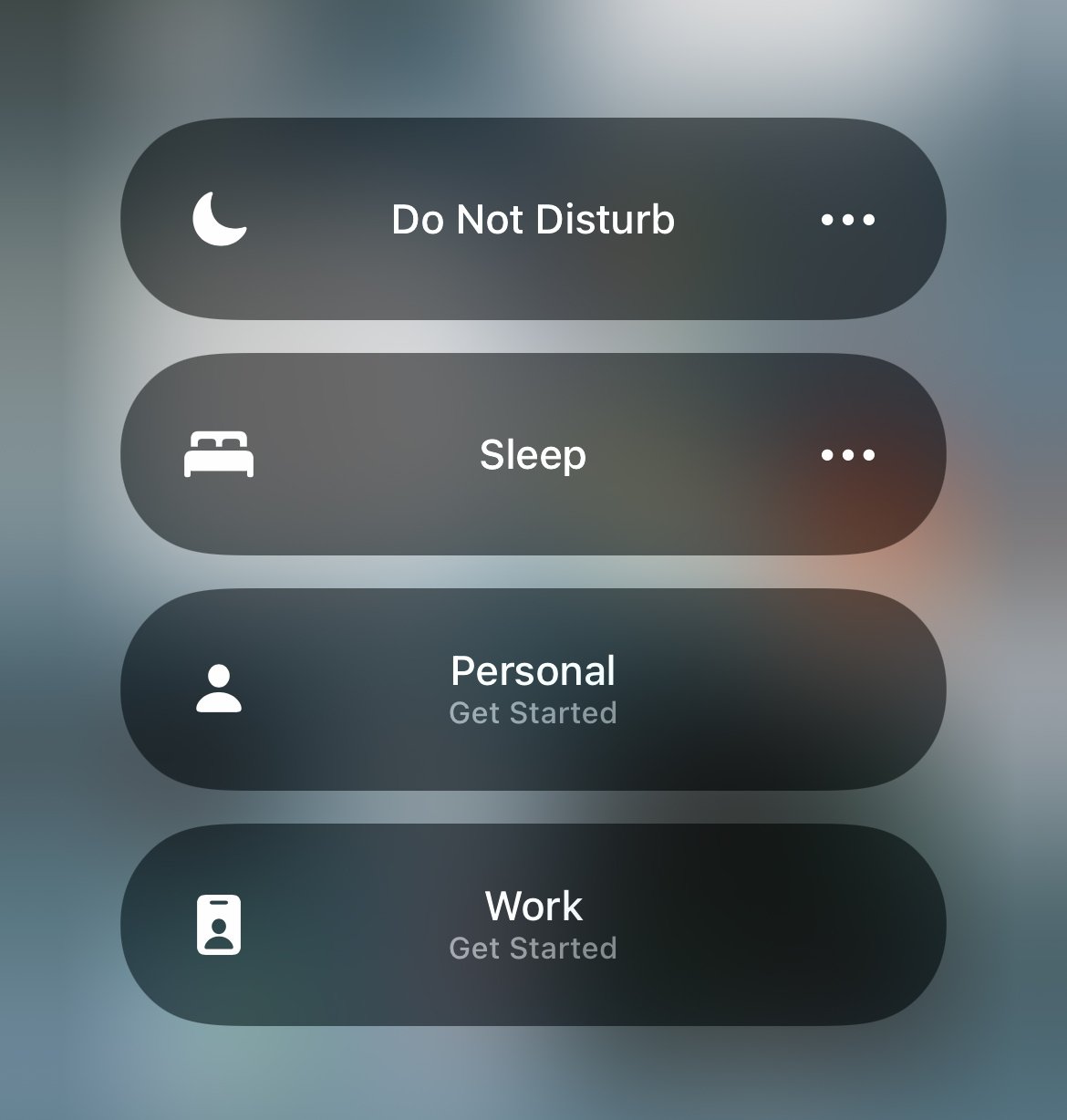The image features a blurry background with hues of black, gray, white, and a touch of orange on the right side. There are four prominently displayed black ovals, each containing distinct white symbols and text. 

The first oval on the left showcases a white crescent moon, accompanied by the text "DO NOT DISTURB" in capital letters. Additionally, three white lines appear in the right-hand corner of this oval.

The second oval depicts a white bed icon with the word "SLEEP" inscribed in the center, also in all capitals. Similar to the first oval, three white lines are present on the right side.

The third oval features an outline of a white figure and bears the text "PERSONAL GET STARTED," all in uppercase letters. The word "PERSONAL" is positioned above "GET STARTED."

The fourth and final oval contains an illustration resembling a badge with a loop at the top, often used with lanyards. The word "WORK" is boldly printed in the center, followed by "GET STARTED" in smaller, white, non-bold text underneath.

Each symbol and text in the ovals is distinct and designed to convey specific messages.